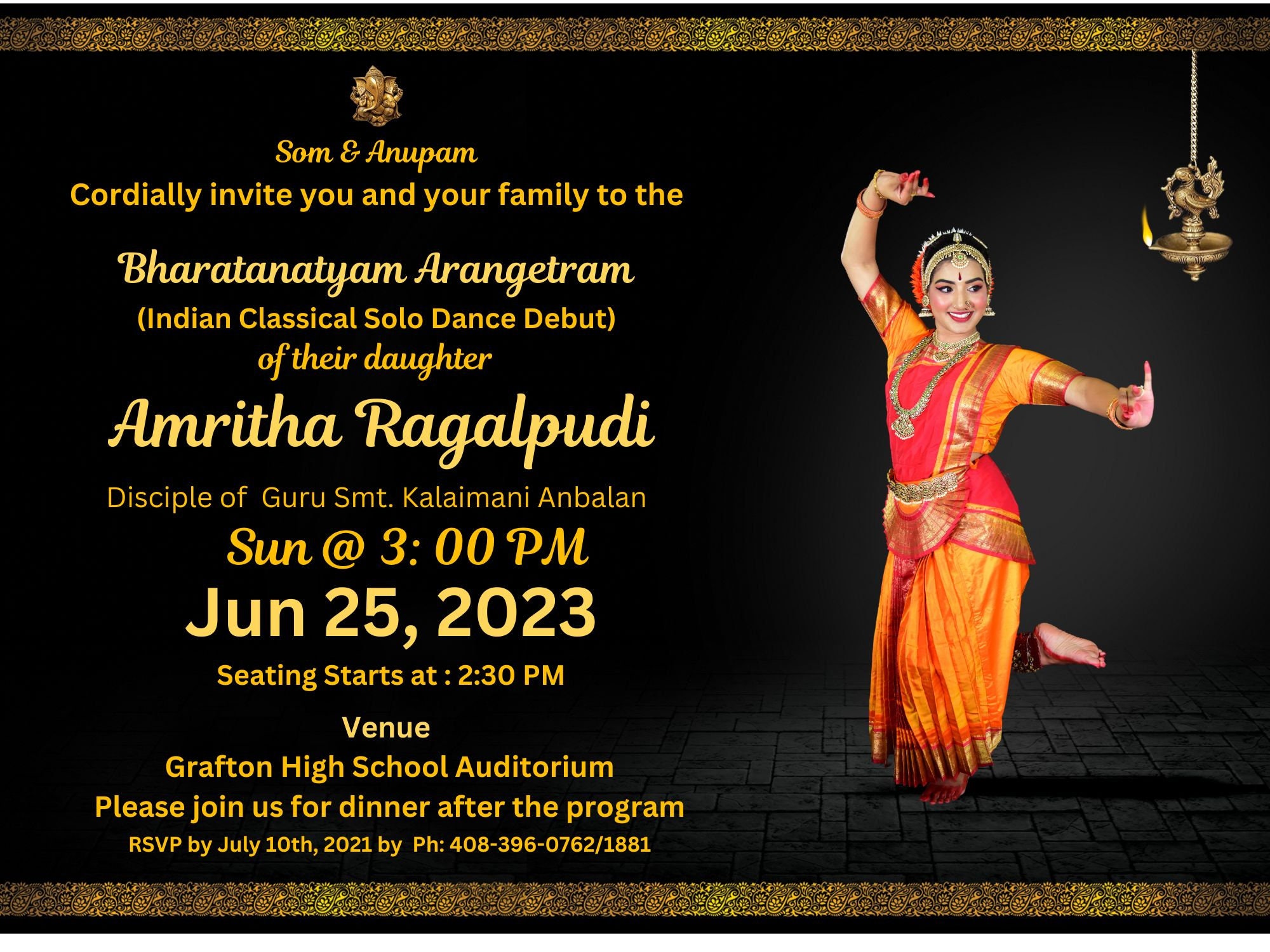The image, set against a black background with dark to charcoal gray gradients and gold borders at the top and bottom, serves as an advertisement for a cultural event. Dominating the right side, the photograph features a woman performing a traditional Indian dance, dressed in an ornate red and orange attire that extends to her bare feet. She displays a graceful dance pose with her right foot lifted behind her, her right arm held above her head, and her left arm extended to the right with her pinky finger raised. Adorning her head is a traditional gold headband with a central tassel, and she's accessorized with gold earrings, a large gold necklace, and bracelets.

Adjacent to the dancer is an ornate hanging lantern, featuring a gold duck perched atop a chain, with a bowl beneath it holding a lit flame. Positioned to the left, the text reads: 

“Som and Anupam cordially invite you and your family to the Bharatanatyam Arangetram (Indian classical solo dance debut) of their daughter, Amrita Raghalpudi, disciple of Guru SMT Kalaimani and Balam. Sunday at 3 p.m., June 25th, 2023. Seating starts at 2:30 p.m. Venue: Grafton High School Auditorium. Please join us for dinner after the program. RSVP by July 10th, 2021, by phone: 408-396-0762 or 1881.”